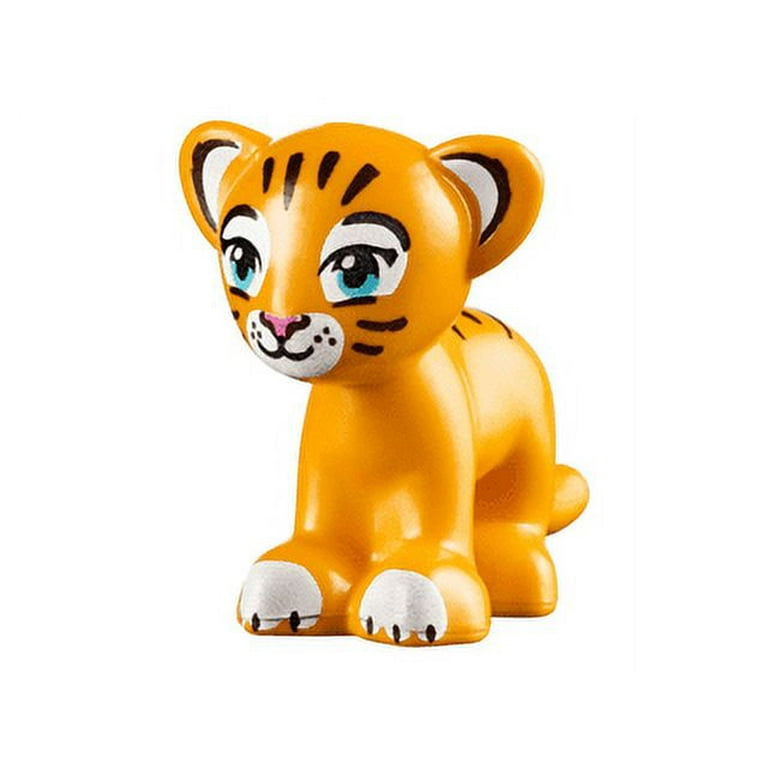In the image, there is a small, goldish-orange plastic figurine depicting a baby tiger. The tiger sits against a pale white background, featuring three stripes on its back and four stripes on its forehead. The face of the figurine is cutesy, with anime-like eyes that are strikingly human-like, outlined with white rings, blue irises, and black pupils. The eyes have feminine cat-eye lines, and the tiger wears a warm smile.

The nose of the tiger is painted pink, with white whiskers extending on either side from a small, white-painted muzzle. The ears are detailed with black borders and white inner coloring. The front paws of the tiger resemble worn shoes with painted white toes and black nails, though mostly obscured. The hind leg appears as a small orange boot. The overall look of the figurine is round and solid, with a cheaply made appearance. The tail is a noticeable nub at the back, completing the charming, whimsical figure.